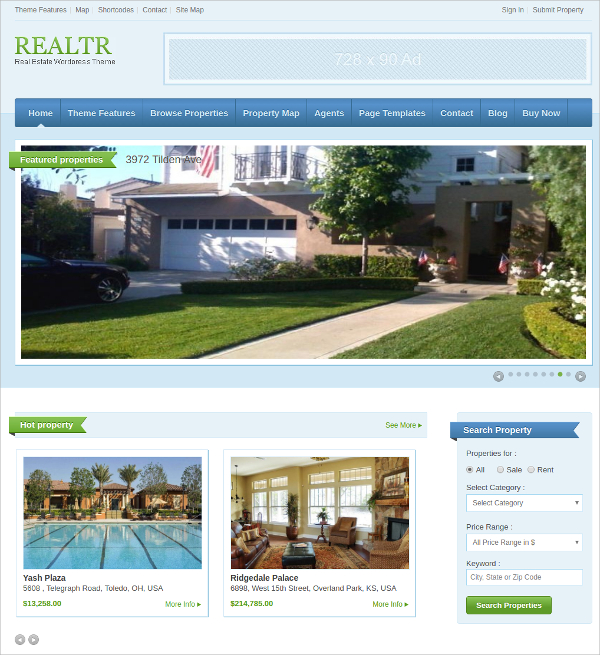Depicted in this image is a highly detailed real estate business webpage designed for a realtor or real estate business team. The top left corner features text outlining the theme, various features, a map, some coding elements, contact information, and a shop map. Moving to the top right, you can find options such as "Sign In," "Submit Property," as well as navigation links including "Home," "Theme Features," "Browse Properties," "Property Map," "Agents," "Page Templates," "Contact," "Blog," and "Buy Now."

In the forefront, prominent imagery displays a house accompanied by a luxurious pool, emphasizing the high-end properties available. Prices are visibly marked, with the first house listed at $13,258 and the second at $214,785.